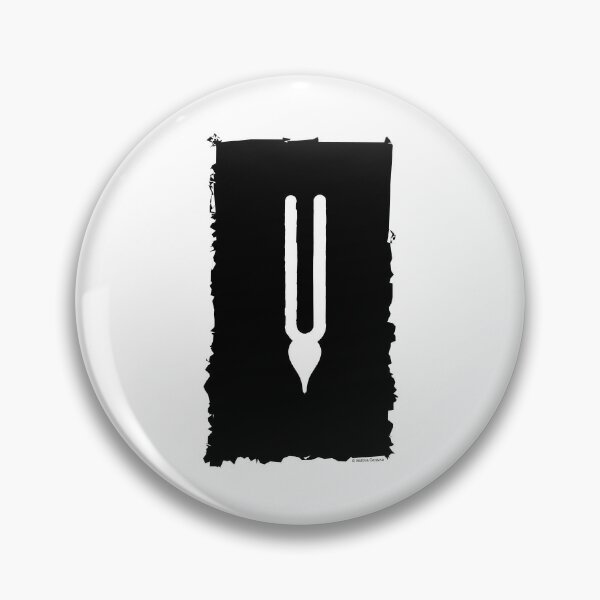The image features a meticulously rendered 3D representation of a white circle set against a stark white background. It appears to resemble a flat white plate, viewed directly from above, seemingly casting a slight shadow for added depth. Dominating the center of the circle is a roughly ink-stamped black box with irregular edges. Inside this black area, a white symbol stands out, bearing a striking resemblance to a tuning fork with an elongated spade handle, or alternatively, an upside-down U with a paintbrush-like head. The overall composition, blending elements of painting and 3D art, creates a visually intriguing interplay of light, shadow, and form.